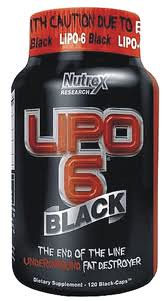This photo features a sleek black canister prominently branded with the "Nutrex Research" label. The container's design is striking, with "Lipo-6" boldly printed in large red letters against the dark backdrop. Just beneath, the word "Black" is emblazoned in matching dark color, creating a visually cohesive look. Lower down, in sharp white text, it declares "The End of the Line Fat Destroyer," underscoring its intense branding message. The canister is topped with a sealed red cap that stands out sharply against the black container, enhancing the overall dramatic effect. Around the top of the cap, a red band mimics caution tape, inscribed with a warning that reads "Open with Caution." Adding to the cohesive branding, "Lipo-6" is also written in white on the cap, completing the container's detailed and cautionary aesthetic.